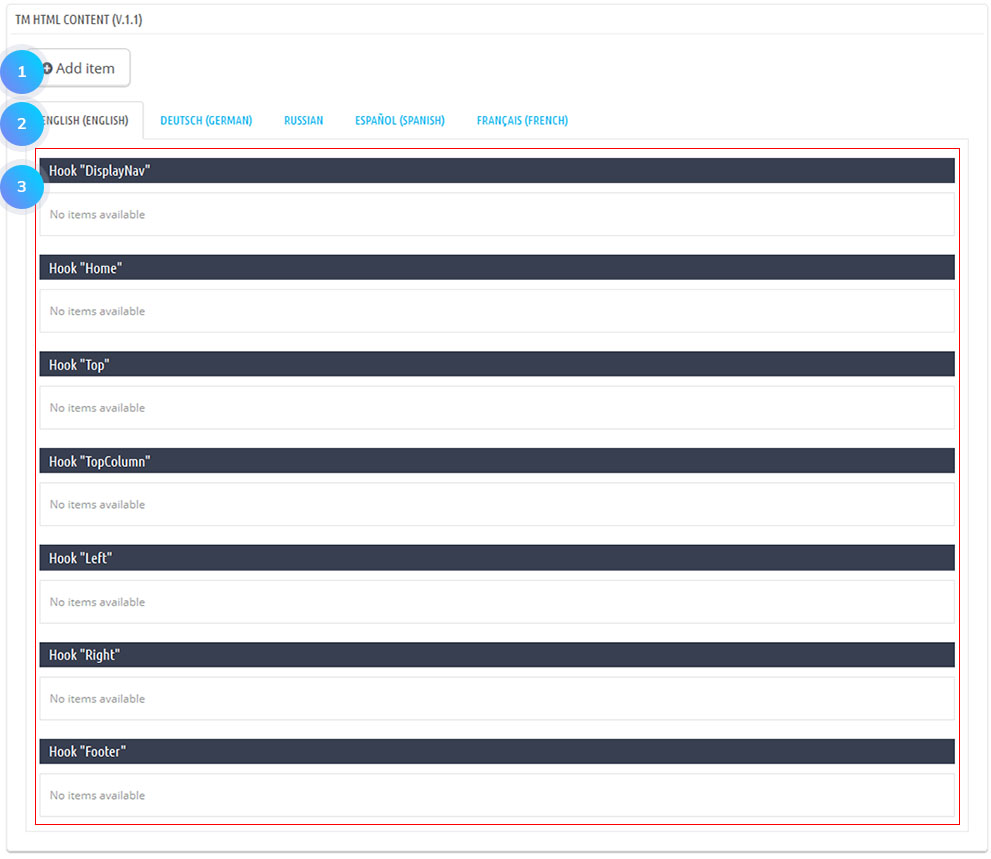The screenshot appears to be from a CAD program designed for home building, though it initially resembles video game commands. At the top right corner of the interface, the text "TM HTML Content Version 1.1" is displayed, indicating the software version. Beneath this is an "Add Item" button, likely used for adding design elements. The program supports multiple languages, including English, German, Russian, Spanish, and French, with English currently selected as indicated by the highlighted option.

In the main section of the interface, a series of black rectangular buttons stretch horizontally across the screen, each containing different command codes in white text. These commands seem to pertain to various structural elements of a house's front facade. The commands include labels such as "Home," "Top," "Top Column," "Left," "Right," and "Footer," which suggest different sections or views of the facade. Overall, the interface provides a detailed set of tools and commands for designing the exterior layout of a home.